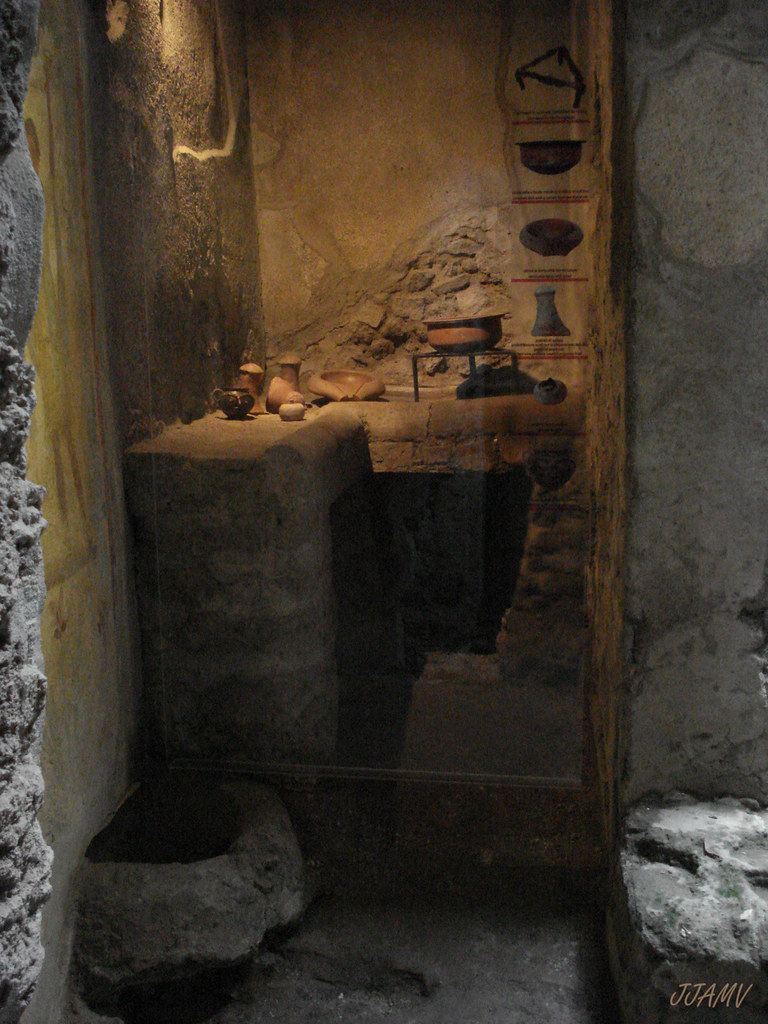The image depicts a museum display set within walls of ancient, weathered stone, suggesting a historical or archaeological exhibit. The stone walls are meticulously aged, giving a sense of authenticity and antiquity. Within the stone enclosure, there's a recessed niche containing the main display, bordered by a wooden frame and protected by glass.

Inside the niche, a stone workstation or table is the focal point, displaying an array of artifacts. These include several bowls, a mortar and pestle, and various jars, all indicative of historical use in domestic or medicinal contexts. Surrounding the glass enclosure are photographs of the displayed objects, with small explanatory text that, while illegible in the image, likely provides context and descriptions for museum visitors. The overall atmosphere suggests a snapshot into an ancient life, preserved and presented for educational purposes.